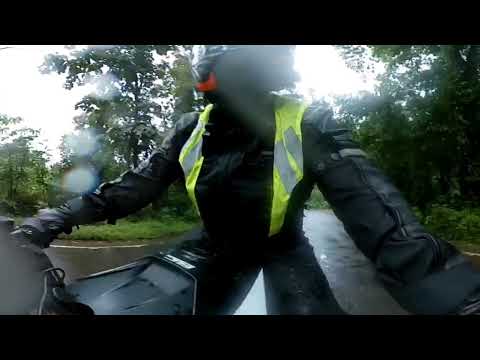The photograph depicts a motorcyclist dressed in full black leather gear, including a black helmet with a red accent near the mouth. The helmet is only partially visible as it extends off the top center of the image. The rider also wears a neon green and silver reflective vest over their jacket, along with black leather gloves. They are straddling a black motorcycle, although only the center console and seat of the bike are visible from this angle. The camera appears to be mounted on the handlebars, aimed towards the driver. The background features dense green foliage and trees, with a light white sky overhead. The road beneath the bike is dark gray and slightly wet, as evidenced by water droplets on the left side of the camera lens. This suggests it may have recently rained, contributing to a cool atmosphere with the sun intermittently shining through the trees.